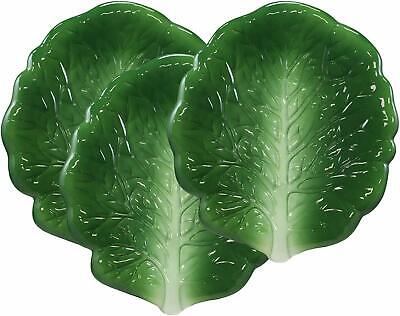The image displays three ceramic platters shaped like vegetable or cabbage leaves, artfully arranged in an inverted pyramid against a stark white background, making them appear as if they are floating. The platters, resembling lettuce leaves with an intricate, jelly-like translucence, are glossy and reflective. Each platter features a central, light-colored vein branching into various sections, enhancing the impression of realism. The platter on the right is fully visible and showcases an elliptical, vertically oriented shape with a scalloped edge. The vivid green color and photorealistic detail suggest they could be carved jade, as they depict different tree and plant patterns etched into the surface. The arrangement and detailed craftsmanship highlight the natural beauty and artistic representation of leaves.